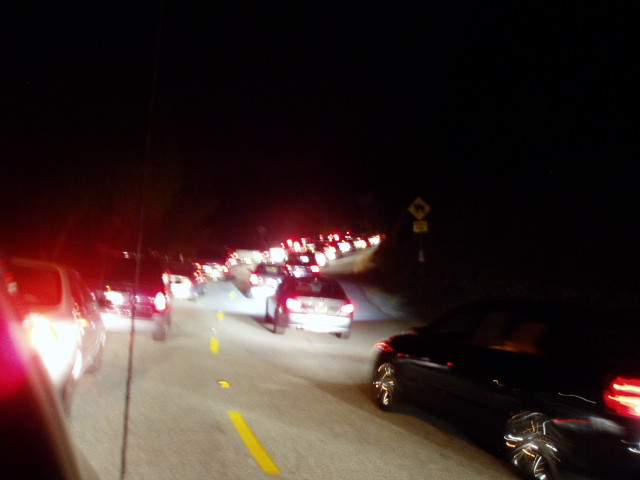This nighttime scene captures a busy stretch of an interchange ramp on a freeway, likely taken from the passenger seat of a car. The road, which is shrouded in pitch black darkness, features two lanes separated by a yellow dashed line with reflectors. The intense glare of countless red taillights illuminates the way, revealing a seemingly endless line of cars and trucks stuck in bumper-to-bumper traffic. The road curves to the middle right of the image, disappearing behind an embankment, giving the impression that it might be merging into another highway.

Notable in the lower left corner is a sleek, black sedan with shiny chrome rims, adding a hint of sophistication to the scene. The gray road below is marked with yellow hash marks, and there's a yellow road sign on the right side, indicating a turning point. The cars appear slightly blurry, emphasizing the impression of the slow, crawling pace typical of rush hour traffic. The top side of the image fades into complete darkness, reinforcing the heavy, sluggish atmosphere of this gridlocked night.